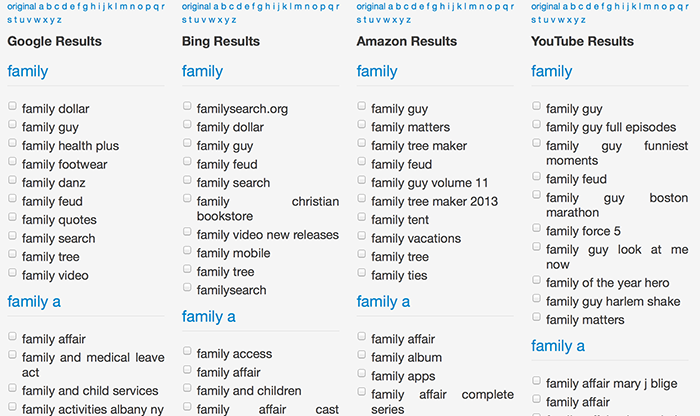This image is a screenshot of a computer display featuring a four-column comparison of search results from different sources. The background is entirely gray, and each column is uniformly labeled at the top. The first row of headers across all columns reads "Original," followed by columns marked as "A," "B," "C," and so on through "Q," "R," and continuing to "Z" on the next line. The columns are titled as follows: the first from the left is labeled "Google Results," the second as "Bing Results," the third as "Amazon Results," and the fourth as "YouTube Results," all written in black text.

Further down the screen, each column features the header “Family” written in blue. Beneath this section, the search results display various phrases related to "family" such as "Family Dollar," "Family Guy," "Family Health Plus," "Family Footwear," "Family Matters," "Family Tree Maker," and "Family Feud."

Moving further down, each column showcases results starting specifically with the letter "A," including terms like "Family Affair," "Family Access," "Family and Children," "Family Album," and "Family Apps." This consistent categorical organization presumably continues for further letters and terms related to the keyword "family."